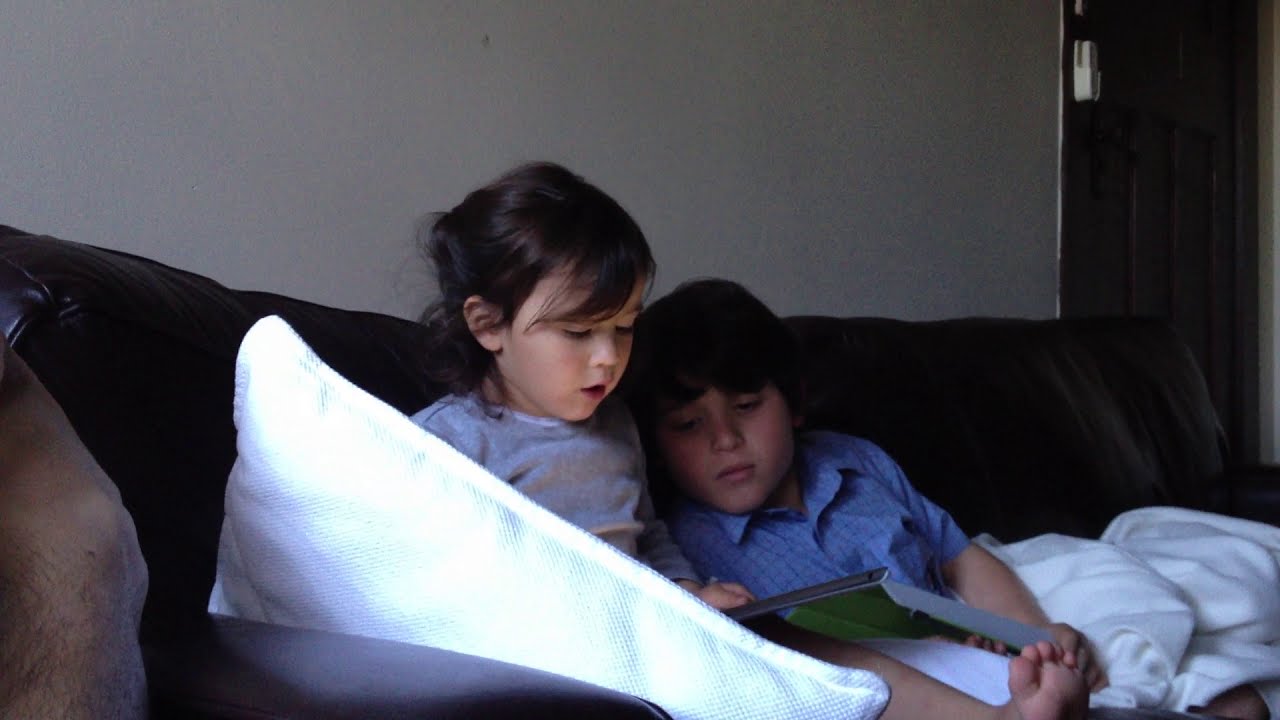In this detailed photograph taken inside a room, two young siblings are warmly nestled together on a brown couch, deeply engrossed in a gray tablet the girl is holding. The brother, who appears to be about three to four years old, has short brown hair and is dressed in a blue collared shirt. His younger sister, possibly around two years old, has darker brown hair and wears a long-sleeved gray shirt. Both children are comfortably enveloped by a soft, white blanket, with a matching white pillow nearby. Their cozy setup is accentuated by the black door visible behind them on the light-colored wall, suggesting a typical domestic setting. The image exudes warmth and sibling bond as both children’s eyes are fixed on the tablet, absorbed in what seems to be a captivating story or game. An adult figure, possibly a parent, is faintly discernible next to them, providing a sense of safe supervision.